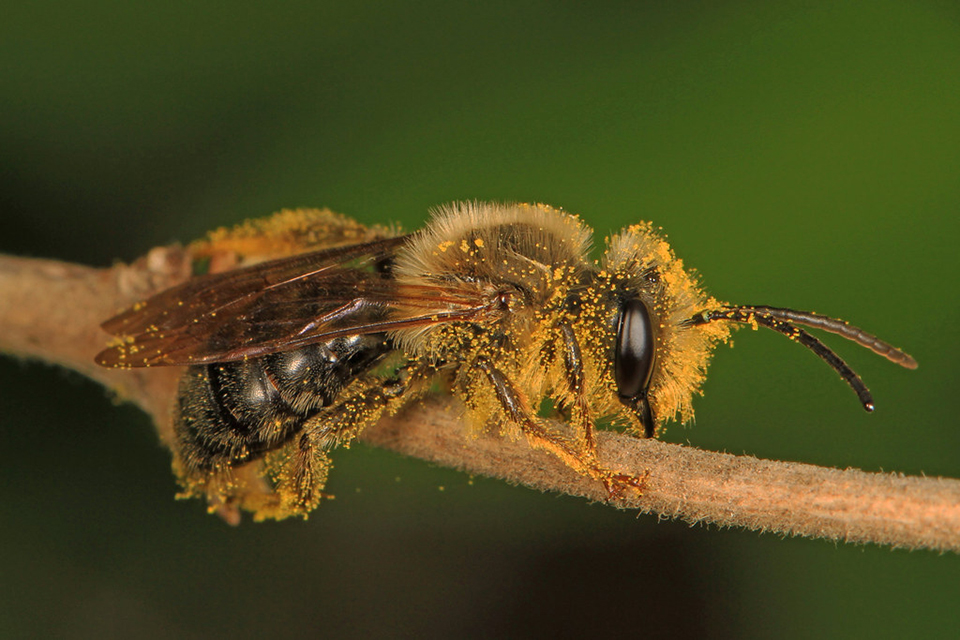This is an extremely close-up photograph of a honeybee, beautifully detailed against a deep jade green background that transitions from darker shades in the bottom left corner to lighter hues in the top right. The honeybee, covered in yellow pollen, is perched on a fuzzy, light brown twig. It features a black body adorned with tufted, creamy yellow fur. The bee's two antennae are black and almost see-through, blending seamlessly with its big, glossy black eyes. The delicate, translucent wings have a light golden-brown tint. The intricate details of the bee's fur and the pollen grains are vividly captured, highlighting the intricate beauty of this small yet important creature.